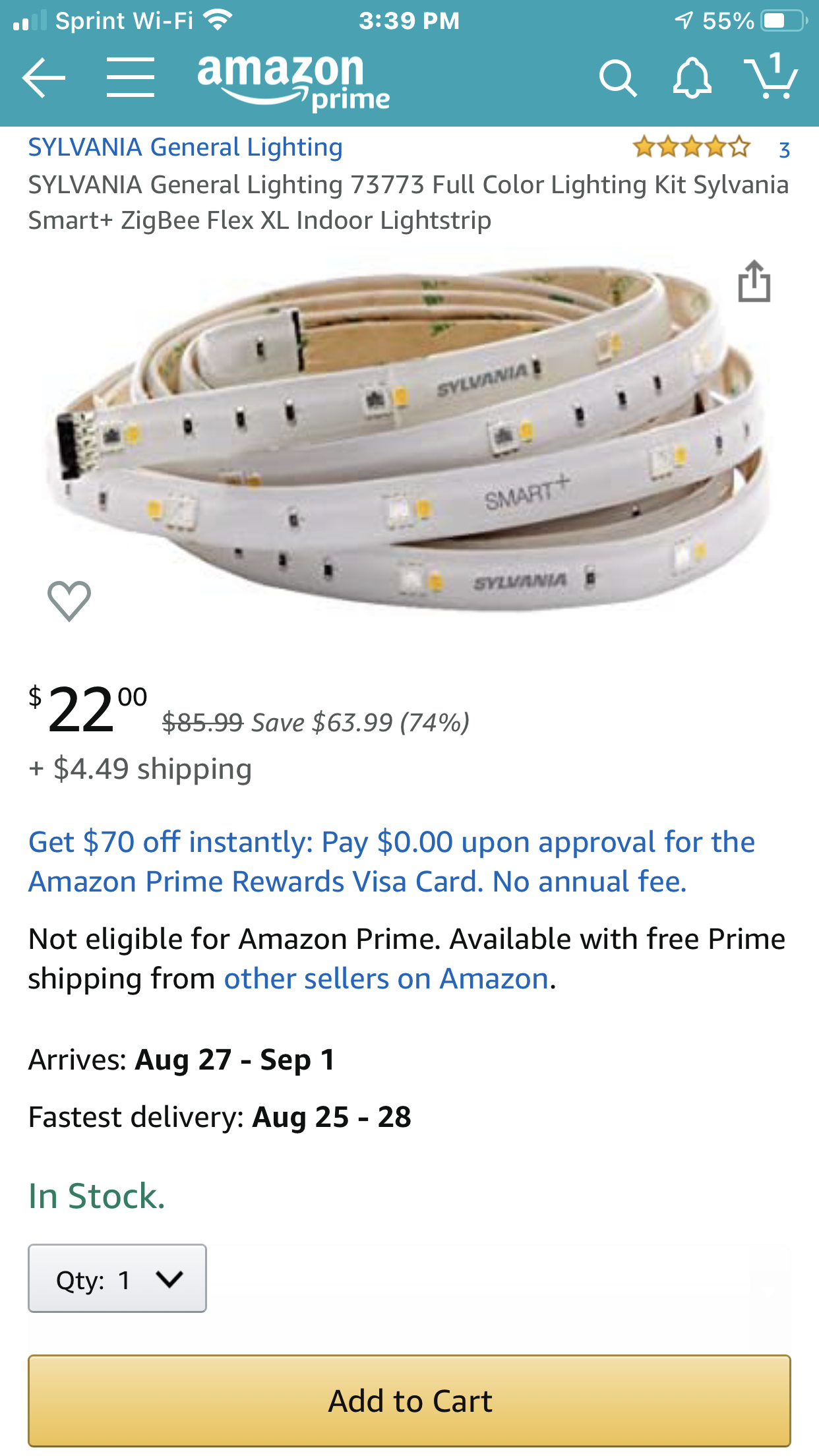This image is a detailed screenshot of an Amazon Prime product page. At the very top of the screenshot, there is a teal banner containing various status icons including cell signal strength, a Wi-Fi signal, the time (3:39 PM), and the battery level at 55%. To the left of these icons, there is a back arrow and three horizontally stacked lines indicating a menu option.

Below the teal banner, the header section contains the Amazon Prime branding and several utility icons: a magnifying glass (search), a notification bell, and a shopping cart displaying the number one inside it.

The main section of the page is set against a white background and begins with a blue text header that reads "Sylvania General Lighting." Adjacent to this header is the star rating for the product, which shows a rating of three stars.

The product title in black text follows, reading: "Sylvania General Lighting, 73773, Full Color Lighting Kit Sylvania Smart Plus Zigbee Flex XL Indoor White Strip." Below the title, there is a product image along with a little heart icon for adding the item to a wish list.

The price is listed as $22.00 plus an additional $4.49 for shipping. Underneath this, a blue text promotion states: "Get $70 off instantly. Pay $0.00 upon approval for the Amazon Prime Rewards Visa card, no annual fee."

Further down, black text indicates that the item is "Not eligible for Amazon Prime," and offers more details about availability: "Available for free Prime shipping from other sellers on Amazon. Price August 27 through September 1st. Fastest delivery August 25th through the 28th."

Finally, there is a dropdown menu for selecting the quantity (defaulting to one) and an "Add to Cart" button.